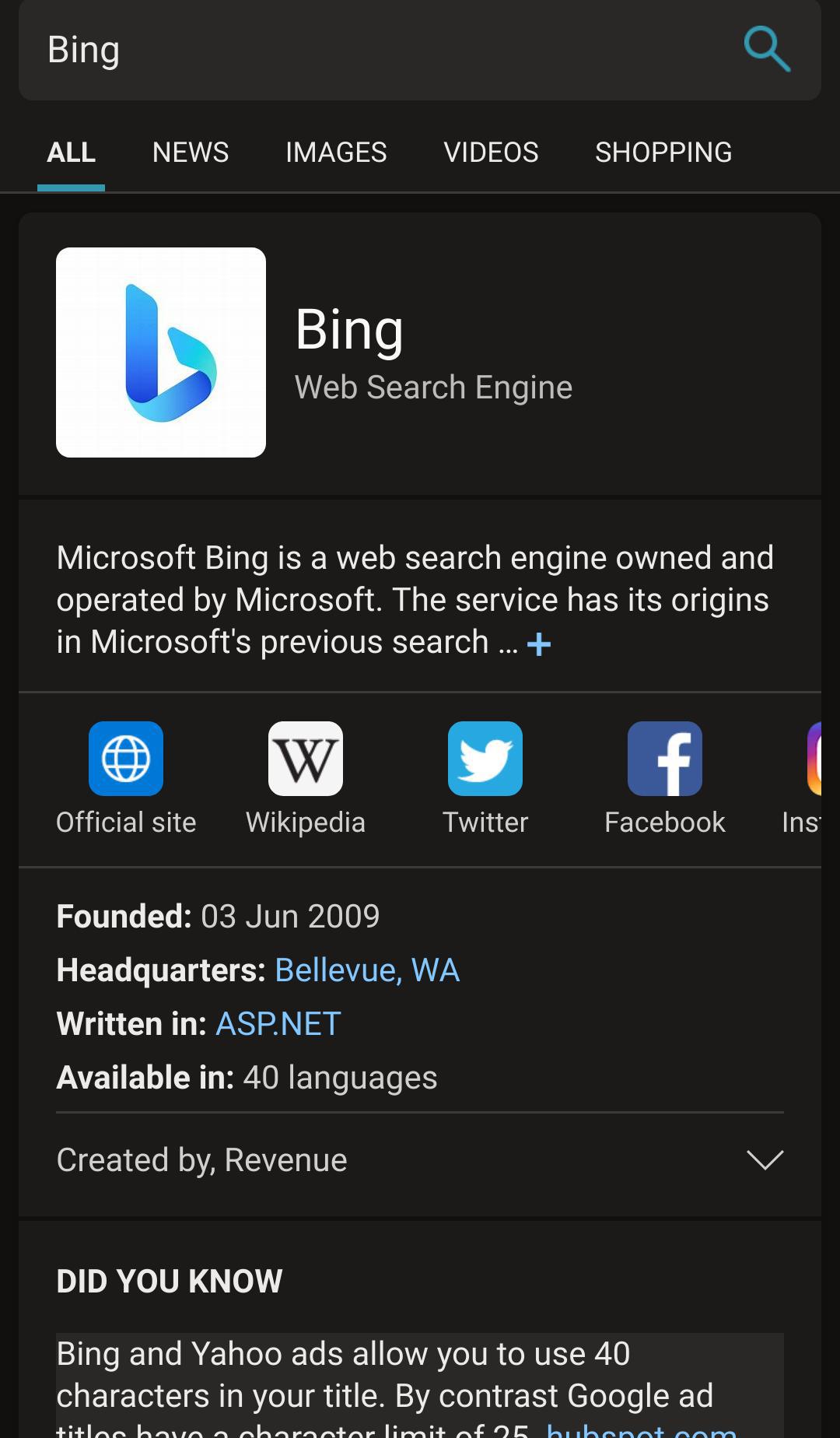The image appears to be a screenshot of a website, featuring a prominent search bar at the top. On the left of the search bar is the Bing logo, displayed in white text. To the right of the search bar, there is a blue magnifying glass icon. Below the search bar, headers in white text are labeled "All," "News," "Images," "Videos," and "Shopping."

The main section of the image showcases the Bing icon, which is depicted as a blue ribbon shaped like a 'B' within a white box. Adjacent to this icon, the text reads "Bing Web Search Engine." Below this text, a brief description states, "Microsoft Bing is a web search engine owned and operated by Microsoft. The search engine has its origins in Microsoft's previous search...". This is followed by a blue plus sign indicating more information.

Further down, there are icons representing different websites: 
- A globe icon labeled "Official Site".
- A large black "W" in a white box for Wikipedia.
- A bird icon for Twitter.
- A white "F" in a blue box for Facebook.

Additional information is provided at the bottom of the section, detailing:
- Founded on 03 June 2009.
- Headquarters located in Bellevue, Washington.
- Written in ASP.net and available in 40 languages.
- Created by Revenue.

There is also a dropdown menu arrow accompanying a fact stating, "Did you know Bing and Yahoo ads allow you to use 2 to 40 characters in your title? By contrast, Google ad titles have a character limit of 25."

The entire website interface is set against a striking black background, which accentuates the white text and colorful icons.